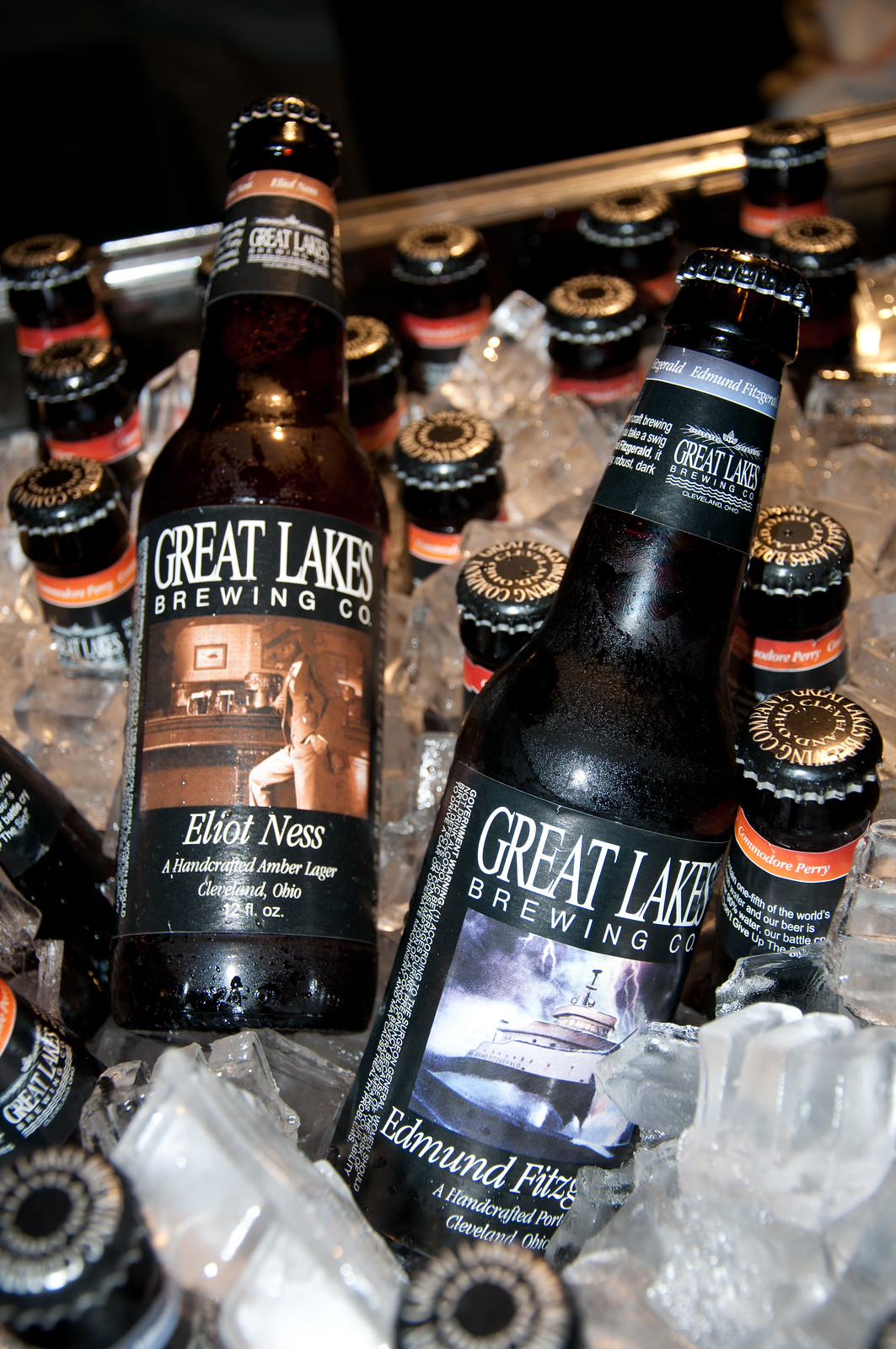The photograph captures a close-up of a stainless steel cooler brimming with ice, showcasing two prominent dark brown bottles from the Great Lakes Brewing Company. The condensation on the bottles indicates that the beer is chilled and ready for consumption. Most of the beer bottles are submerged in ice, with only their necks visible, but two bottles are positioned more prominently.

The bottle on the left features a sepia-toned label with the image of Elliot Ness standing at a bar. Beneath the image, the label reads: "Elliot Ness, a handcrafted Amber Lager, Cleveland, Ohio, 12 fluid ounces." The label has a distinct brownish hue that compliments the amber color of the beer within.

The bottle on the right showcases a black-and-white image of a ship battling a stormy sea, with large swells, beneath which it says: "Edmund Fitzgerald, a handcrafted," with part of the details obscured by the ice. The label of this bottle has a blue tint, enhancing the maritime theme.

Together, the photograph captures the rustic and crafted appeal of the Great Lakes Brewing Company's specialty beers, encapsulated in a cool, inviting scene.